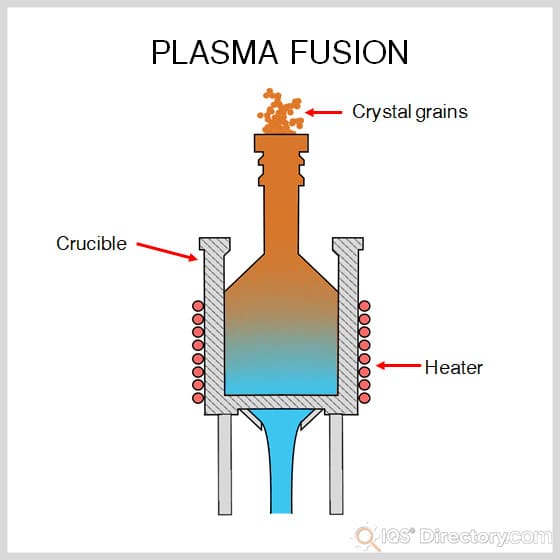This detailed infographic titled "Plasma Fusion" visually explains the process through a series of labeled elements and vibrant colors. Set against a clean white background, the central image closely resembles a science textbook diagram or a slideshow for educational purposes.

At the core of the image lies a crucible, depicted in gray, with its contents illustrated in a gradient of colors. The bottom part of the crucible starts with a sea blue hue that transitions to a rust color as it moves upward, simulating a temperature gradient. This color shift symbolizes the heating process, with the blue representing cooler temperatures and the rust color indicating higher temperatures.

The infographic includes three main labels, each indicated by a red arrow. At the very top, "Crystal Grains" is marked with an arrow pointing to a section at the pinnacle of the crucible, where small orange dots appear, likely representing the formation of grains through plasma fusion. The "Crucible" label is positioned toward the middle, with its arrow pointing to the gray container itself. On the right side, "Heater" is designated, with a red arrow leading to a series of circles aligned vertically along the crucible's exterior, illustrating the heating mechanism applied externally to achieve fusion.

Subtle intricacies, such as the hourglass-shaped logo bearing the text "iqsdirectory.com" at the bottom and a depiction of something molten fusing within the crucible, add layers of context to the illustration. The image incorporates smooth visual flows and detailed points of interest to describe the transformation process during plasma fusion, aimed at fostering a comprehensive understanding of the phenomenon.